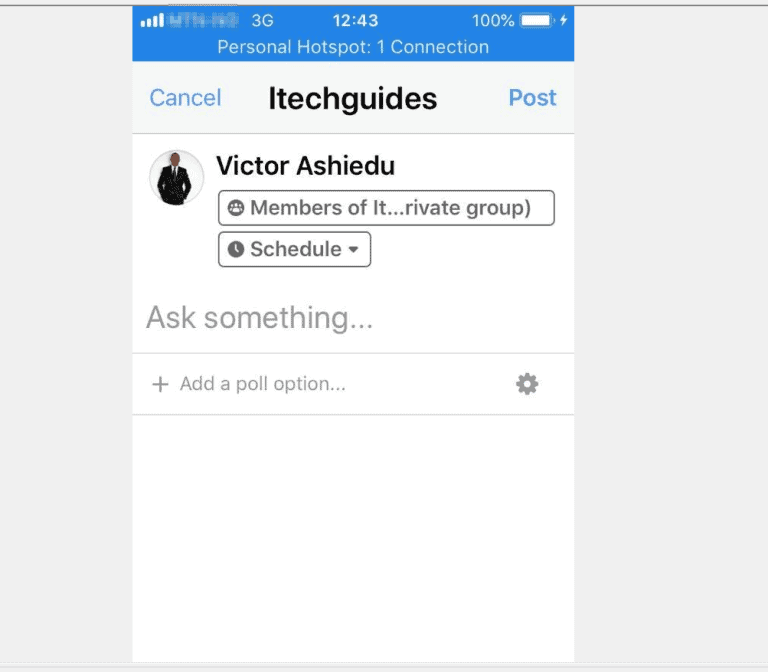A smartphone screen displaying a Wi-Fi connection with full signal, a 3G network, and a fully charged battery at 12:43 (AM or PM), likely while charging. The device is set up as a personal hotspot, currently supporting one connection. The user appears to be engaged with a website called "iTech Guides," which offers advice and support for tech-related questions. At the top of the screen, there are options to either "Cancel" or "Post," both highlighted in blue, indicating these actions are available for the user. The profile picture of Victor Ashidu, a member of the iTech Guides private group, is visible along with his schedule dropdown menu, suggesting he could be available to answer questions. Below, there's an input field labeled "Ask something," accompanied by a plus sign to add a poll option, allowing users to inquire about common issues and receive feedback from others. A settings toggle icon is also present, providing access to additional configurations.